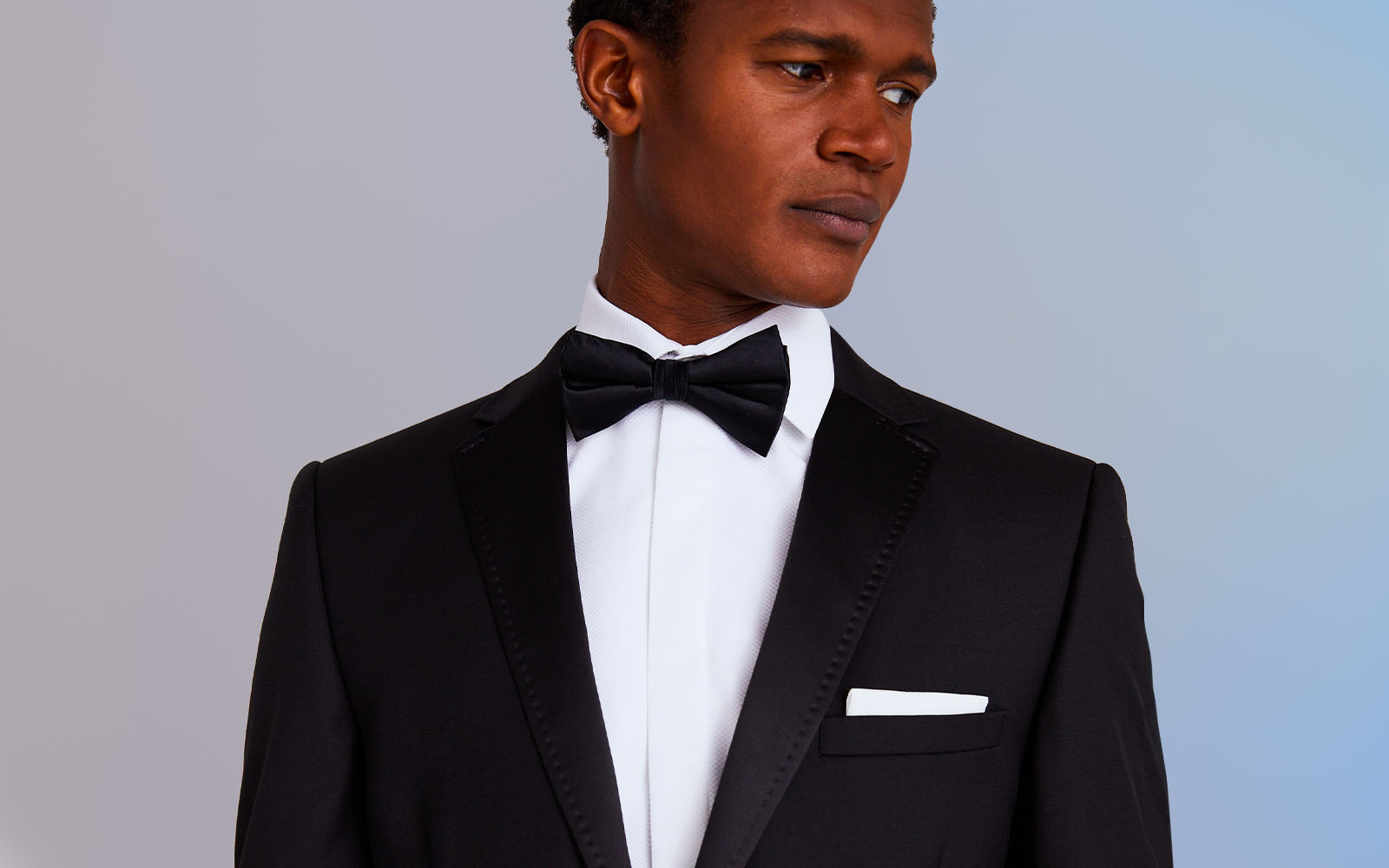This horizontally aligned rectangular photograph features an African American man with very dark skin, depicted from his mid-forehead down to just below his chest. The man's head is tilted to his left (our right) and he's gazing downward. He is dressed in a classic black tuxedo comprising a black bow tie, a white button-down collared shirt, and a black suit jacket with shiny lapels. A neatly folded white pocket square is tucked into the breast pocket on his left side. His hair, which is short and black, gives way to his smooth skin, and he appears to be in his 30s or 40s. The background transitions seamlessly from a solid gray on the left to a solid blue on the right, creating a smooth gradient effect. The man's facial features include broad nose and full lips, and he exudes an aura of elegance and sophistication.